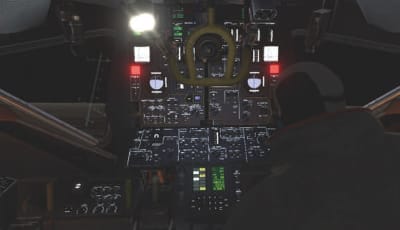The image depicts a dimly lit airplane cockpit, likely photographed at night, with characteristic low visibility. The focal point of the picture is the array of illuminated dials, buttons, and panels, predominantly in shades of gray and black. Central to the console are various controls, including black switches and a notable green display towards the bottom center. The top center features a bright light or possibly a camera, which emits light waves across the cockpit. On the upper left and right, there are striking white and red light squares. A person, potentially a pilot wearing a white helmet and a thick green jacket, seems to be situated on the right, facing away from the camera. The external view through the cockpit windows is dark, suggesting it's nighttime or depicting an otherworldly scene, adding a dreamlike quality to the photograph. The image is not of high resolution, being somewhat grainy and blurry, which contributes to the challenge of discerning finer details but enhances the mysterious ambiance.